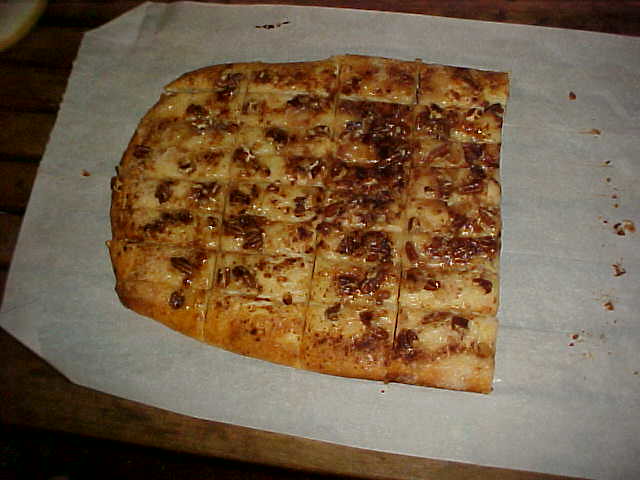This image captures a rustic scene with a wooden tray serving as the backdrop. Dominating the center of this indoor setting is a piece of wax paper, neatly placed on the tray. At the heart of the composition lies a sectioned loaf of bread, which could easily be mistaken for pizza dough due to its appearance. The bread is segmented both vertically and horizontally, with uneven, rounded edges indicating the original, larger shape of the loaf. The browning on top suggests a perfectly baked crust, adorned with what looks to be a scattering of bacon bits. Crumbs are scattered around, forming a semi-circle, implying that a portion of the bread is missing. The image's color palette includes shades of black, brown, light brown, white, yellow, and tan, adding to the rustic and warm ambiance. The scene suggests either a kitchen or a restaurant environment, though the exact location and time of day remain indistinct.